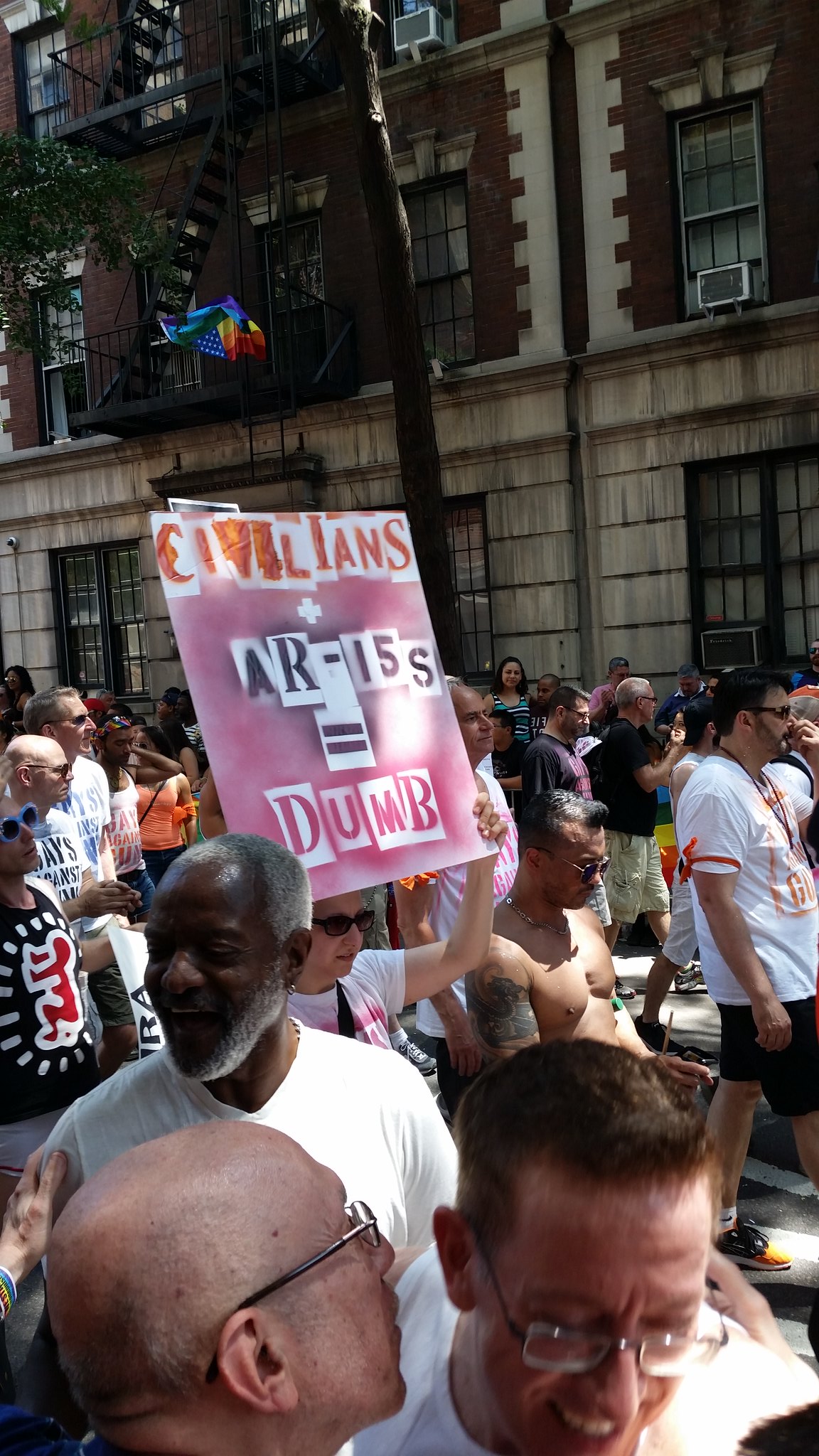The photograph captures a vibrant protest scene, featuring a diverse crowd of people marching down a city street, with a mix of ages, genders, and races, though there are notably more men than women. Prominently visible in the photo is a hand-designed, pink sign held by a woman in sunglasses, which reads in a vertical layout: "civilians + AR-15s = dumb," clearly indicating an anti-gun, specifically anti-assault rifle sentiment. In the background, an apartment building with tall, thin windows and an exterior fire escape system reminiscent of New York City stands out, its upper stories revealing brickwork. Adding to the scene, a rainbow flag with 50 stars, blending the themes of LGBTQ+ pride and American identity, hangs on the building. Among the crowd, two men are seen in a close, supportive gesture, with one man having his arm around the other and whispering in his ear, enhancing the sense of community and solidarity in the protest.